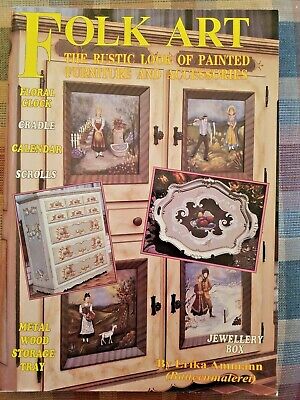The image is a photograph of an old-fashioned book cover titled "Folk Art: The Rustic Look of Painted Furniture and Accessories" by Erika Ammann, also labeled "Buttermalerei." The cover, in bold yellow text, highlights various folk art items such as a floral clock, cradle, calendar, scrolls, metal wood, storage tray, and jewelry box. Centrally featured is an ornate jewelry box with intricate paintings and paneling on its doors, complemented by several drawers. Additionally, two smaller overlaid images present another wardrobe and a serving tray, all set against a backdrop that suggests a kitchen tablecloth. The cover's graphic design appears cluttered, yet it effectively conveys the book's content on traditional, rustic folk art.